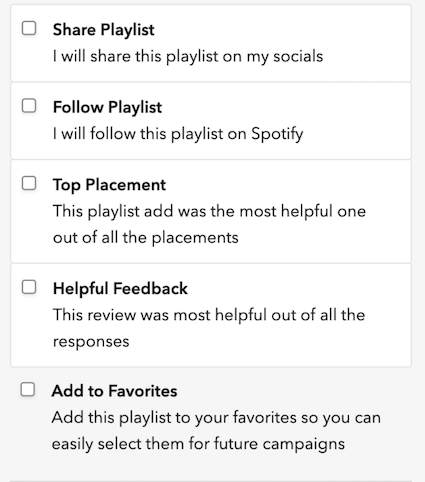The image is a screenshot that appears to be from a mobile application, featuring five distinct rows, each with an option checkbox next to the title. The top row is labeled "Share Playlist," allowing users to share their playlists on social media platforms. The second row is titled "Follow Playlist," providing the option to follow a playlist on Spotify. Each row presents a clear and simple interface for managing playlist interactions, likely through checkboxes that can be toggled. The overall design seems to focus on straightforward user choices for playlist engagement.